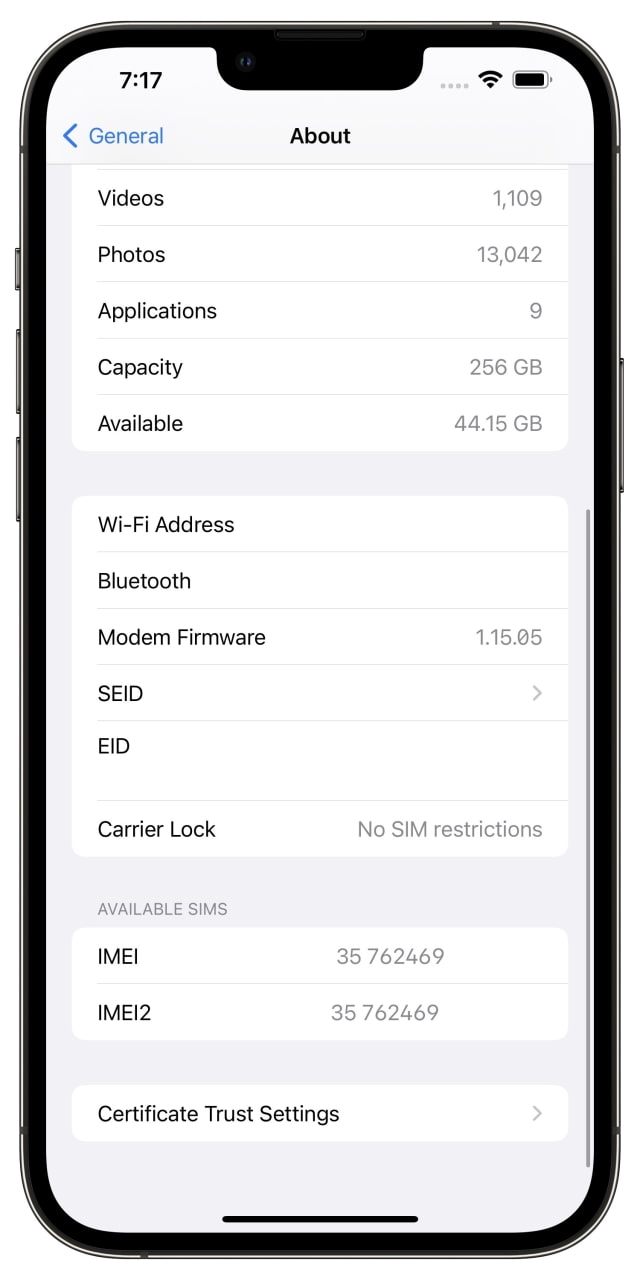The image depicts a cell phone with black edges and clearly visible side buttons. The screen is predominantly white, displaying the time "7:17" in the top left corner. Various status icons are visible at the top right, including symbols for Wi-Fi, cellular signal strength (represented by dots), and a full battery.

On the left side of the screen, a blue label specifies "General" next to a left arrow. In the center, the word “About” appears in black text. Below this, a left-justified list provides detailed information about the phone’s contents and specifications:

- Videos: 1,109
- Photos: 13,448
- Applications: 9
- Capacity: 256 GB
- Available: 44.15 GB

Further down, additional data fields include:

- Wi-Fi Address
- Bluetooth
- Modern Firmware: 1.15.05
- SEID with an arrow directing to the right
- EID
- Carrier Lock: No SIM restrictions
- Available SIMs
- IMEI: 35762469
- IMEI 2: 35762469
- Certificate Trust Settings with another arrow pointing to the right

Each item on the list is separated by a horizontal gray line, and all numerical data align to the right. At the bottom of the list, there is a black line or bar.